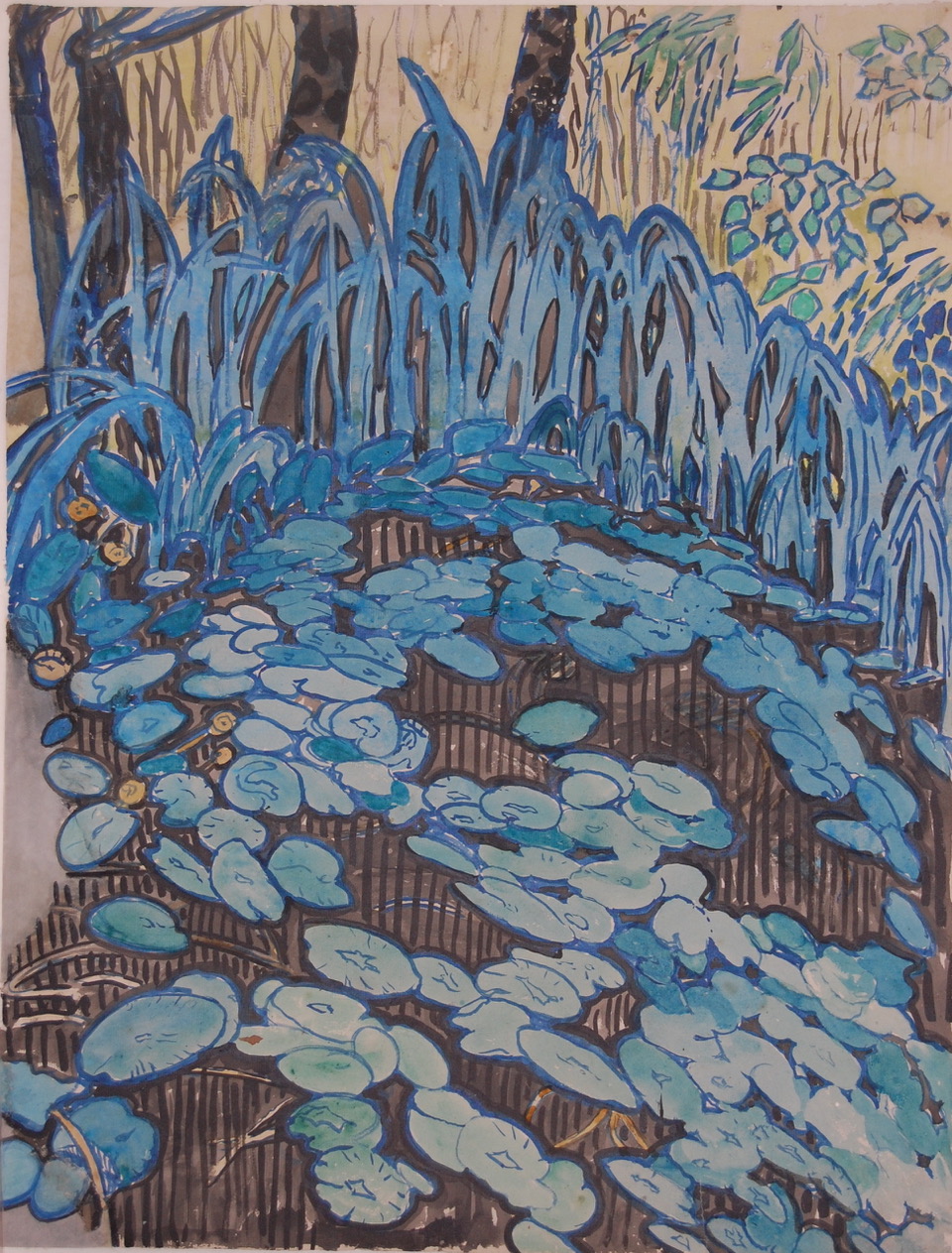This painting, possibly an abstract oil or pastel piece, captures a serene natural landscape. Dominated by hues of blue, it reveals blue waterlilies and petals in the foreground amidst a body of water, possibly a pond, set against a beige backdrop. Surrounding the water are tall, bluish-green reeds that ripple around the edges. The background features slender, brown and black tree trunks interspersed with bluish and yellowish reeds, as well as discreet ferns. This vertical composition evokes the essence of a garden or wild meadow, with patches of brown grass peeking through, creating a layered and textured depiction of nature's quiet, untouched beauty.